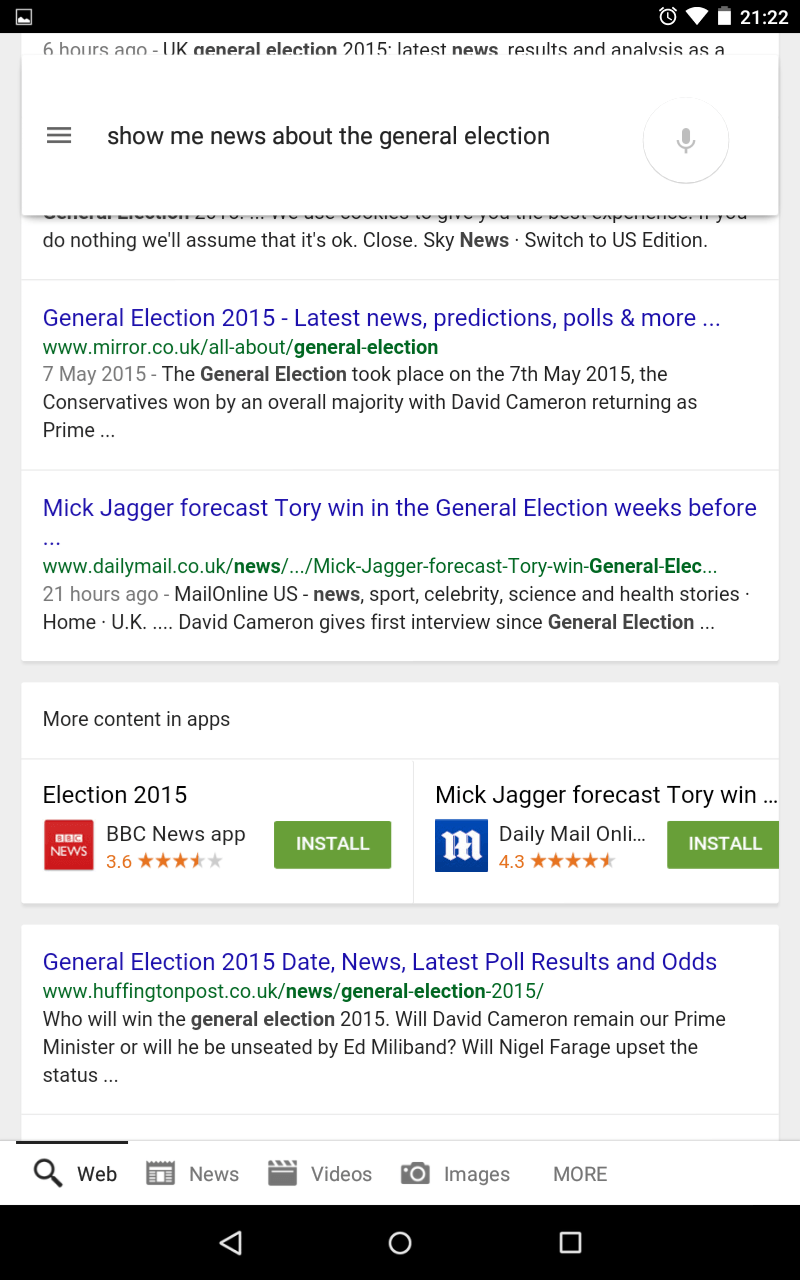**Screenshot Detail of Google Search Results on a Mobile Device for "News About the General Election"**

This image depicts a screenshot of a Google search results page displayed on a mobile device. At the top, there's a black header featuring several icons: a white picture icon to the far left, followed by a white clock icon, a white Wi-Fi icon, a white battery icon indicating a nearly full charge, and the time displayed as '21:22', all situated to the far right.

Beneath this header lies a prominent white search bar. To the left of the search bar is an icon with three horizontal lines, suggesting a menu. The text within the search bar reads, "Show me news about the general election." Adjacent to this text, on the right side of the search bar, is a white circle with a light gray outline encompassing a light gray microphone icon, indicating a voice search option.

The search results are displayed below the search bar. Each result features a header in blue text, a URL in green text, and a brief snippet of information in gray text from the corresponding website. The detailed breakdown of the search results is as follows:

1. **First Result:**
   - **Header:** "General election 2015: latest news, predictions, polls, and more..."
   - **URL:** "www.mirror.co.uk/all-about/general-election-7-May-2015"
   - **Snippet:** "The general election took place on the 7th May 2015. The Conservatives won by an overall majority, with David Cameron returning as prime..."
   
2. **Second Result:**
   - **Header:** "Mick Jagger forecast Tory win in the general election weeks before..."
   - **URL:** "www.dailymail.co.uk/news/.../Mick-Jagger-forecast-Tory-win-general-elect..."
   - **Snippet:** "Mail Online, U.S. news, sports, celebrity, science, and health stories, home, U.K...."

3. **Third Result:**
   - **Header:** "David Cameron gives first interview since general election..."